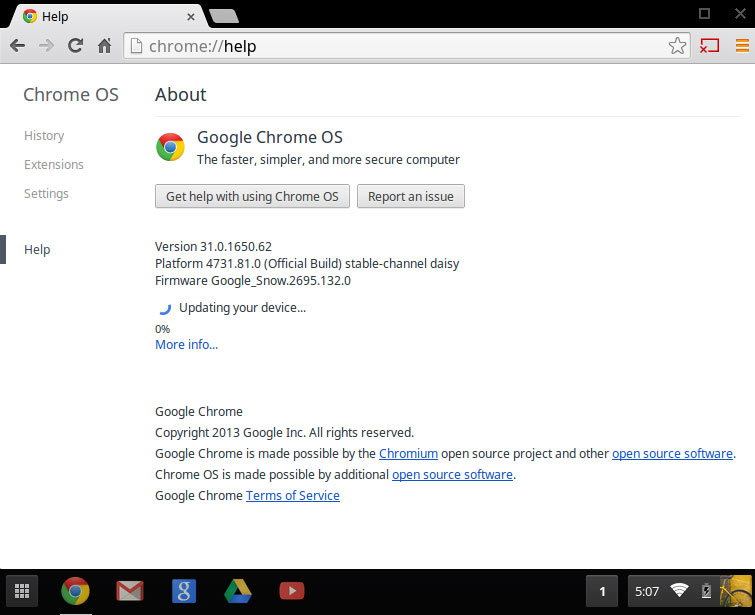The screenshot displays the Google Chrome browser interface. In the upper left corner, the "Help" section is highlighted, with the Chrome logo to its left and a gray "X" button to its right. This is the only tab open in the browser. Below the tab bar, the address bar displays "chrome://help," followed by a star icon and a red rectangular icon with a small red "X" at the bottom left corner. 

To the right of the address bar, there is a vertical ellipsis (three stacked orange lines) which represents the settings menu. Next to it, the window control buttons are visible, including the "Maximize" and "Close" (X) buttons.

The main content of the page is related to Chrome OS, featuring navigation options like "History," "Extensions," "Settings," and "Help," with the "Help" section currently active, as indicated by the vertical dark gray bar on its left. The header reads "About Google Chrome OS: The faster, simpler, and more secure computer."

Below the header, two gray buttons are present: one labeled "Get help with using Chrome OS" and the other "Report an issue." Detailed version information is provided, stating "Version 31.0.1650.62, Platform 4731.81.0 (Official Build, stable channel daisy)," and firmware version "google_snow.2695.132.0."

A status message at the bottom indicates an ongoing update process: "Currently updating your device: 0%." The phrase "more info" is a hyperlink, distinguished by its blue color.